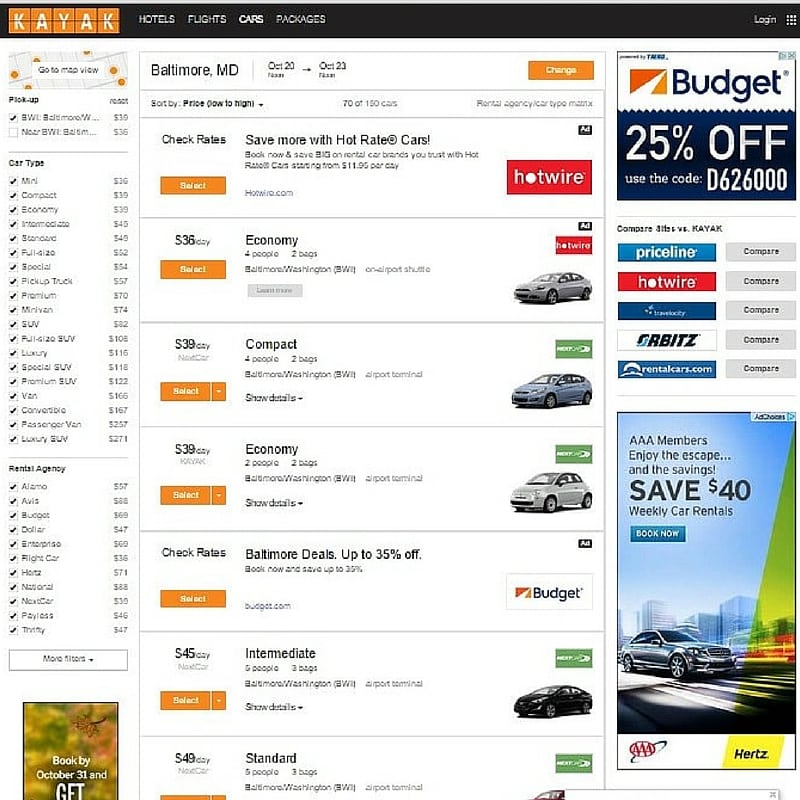The image depicts a webpage from Kayak.com, specifically the section for rental cars in Baltimore, Maryland, covering the rental period from October 20th to October 23rd. The upper part of the image features the navigation bar, prominently displaying the Kayak logo in white letters on an orange background. The navigation options listed in white are Hotels, Flights, Cars (bolded to indicate the active page), and Packages.

On the left side of the main section, there's a sidebar with options for filtering results by location (BWI Airport), car type, or rental agency. Just beneath this sidebar, a portion of an advertisement is visible. The main section of the page, occupying approximately 80% of the image, lists rental car options for Baltimore, Maryland, for the specified dates. The displayed vehicles are organized in five rows, interspersed with advertisements.

1. The top row starts with an ad for Hotwire, followed by an economy car available at $36 per hour.
2. The second row features a compact car at $39 per hour and an economy car also at $39 per hour, followed by an ad for Budget car rental.
3. The next row highlights an intermediate vehicle at $45 per hour.
4. Additional ads are interspersed throughout the list, including a square advertisement on the right side offering 25% off from Budget rental cars.

There are also buttons provided for comparing Kayak's rental car prices with those from other rental companies. This detailed layout helps users efficiently browse and compare rental car options for their trip to Baltimore.